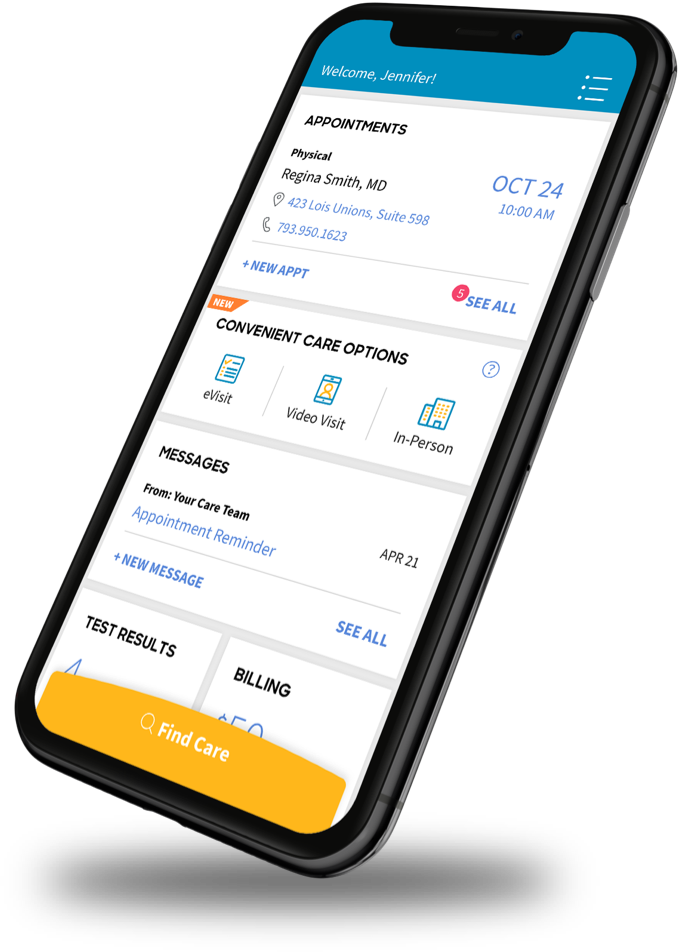The image features a smartphone encased in a black protective cover. The screen displays a user interface, starting with a light blue banner at the top that reads "Welcome, Jennifer" in white text. To the right of this greeting, there is a menu icon consisting of three horizontal bars.

Beneath the banner, on a white background, is a detailed section labeled "Appointments." Within this section, there is an upcoming appointment listed as follows:
- **Physical with Regina Smith, MD**
- **Location:** 423 Lewis Union, Suite 598
- **Phone:** 793-950-1623
- To the right of this information, the date and time of the appointment are displayed: **October 24th, 10 a.m.**

Immediately below this appointment information, there is a button with a plus sign labeled "New Appointment" on the left. To the right of this button, there is a circular icon with the number 5 inside it, which likely indicates notifications or tasks.

Further down, a section titled "Convenient Care Options" is presented with three choices:
- **E-Visits** (on the left)
- **Video Visits** (in the center)
- **In Person** (on the right)

Each of these options features an accompanying icon that visually represents the respective service type.

Below the care options, there is a "Messages" section in black text from the user's care center, with an appointment reminder dated **April 21st**. Adjacent to this message, to the right, is a plus sign for composing "New Messages," along with a circular seal icon.

At the bottom of the screen, the interface is divided into two boxes:
- **Test Results** (on the left)
- **Billing** (on the right)

Finally, the very bottom of the screen features a search bar with the placeholder text "Find Care" alongside a magnifying glass icon on the left, indicative of a search function.